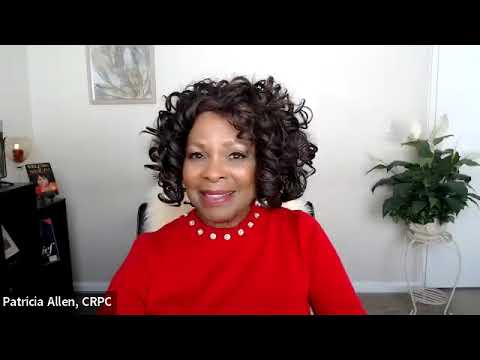The image depicts Patricia Allen, CRPC, an African-American woman with chin-length curly hair, brown eyes, pink lips, and a bright smile that reveals the white of her teeth. She is wearing a red long-sleeved sweater adorned with white dots around the neckline, resembling a necklace. The background features a white wall accented with artwork—a framed sketch of vegetation in a brown frame—positioned at the top left. On the right side, there is a plant with large green leaves placed on a white stand, which casts a shadow on the wall behind it. Additionally, there is a piece of black furniture, likely a desk or shelving unit, on the left side, holding a lit candle with a pink-red hue. In the bottom left corner of the image, her name and credentials are displayed in white text: "Patricia Allen, CRPC."